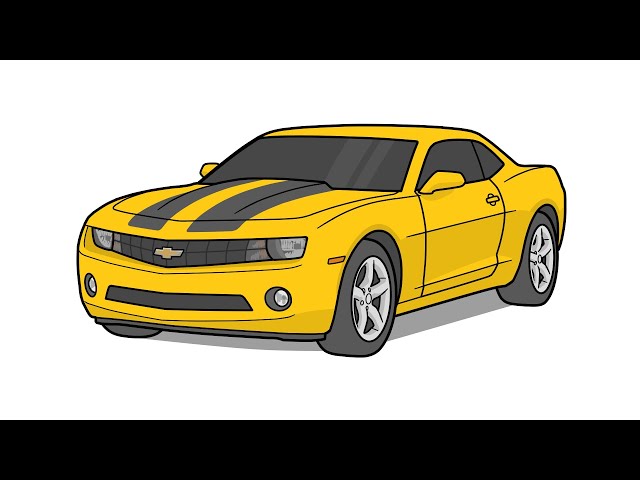This horizontally aligned, rectangular animated image features a yellow Chevrolet sports car centered against a white background. The image is flanked by thick black borders at the top and bottom, creating a framed effect. The car itself is vividly detailed with distinct black outlines, boasting two wide dark gray racing stripes running from the windshield down the hood. It features a tinted black windshield and driver's side windows. The front grill displays the iconic gold Chevrolet emblem, flanked by two small floodlights and a lower, secondary black grill. The car rests on black wheels with silver rims, and subtle shadows accentuate its modern design, enhancing the animated, cartoonish aesthetic of the image.